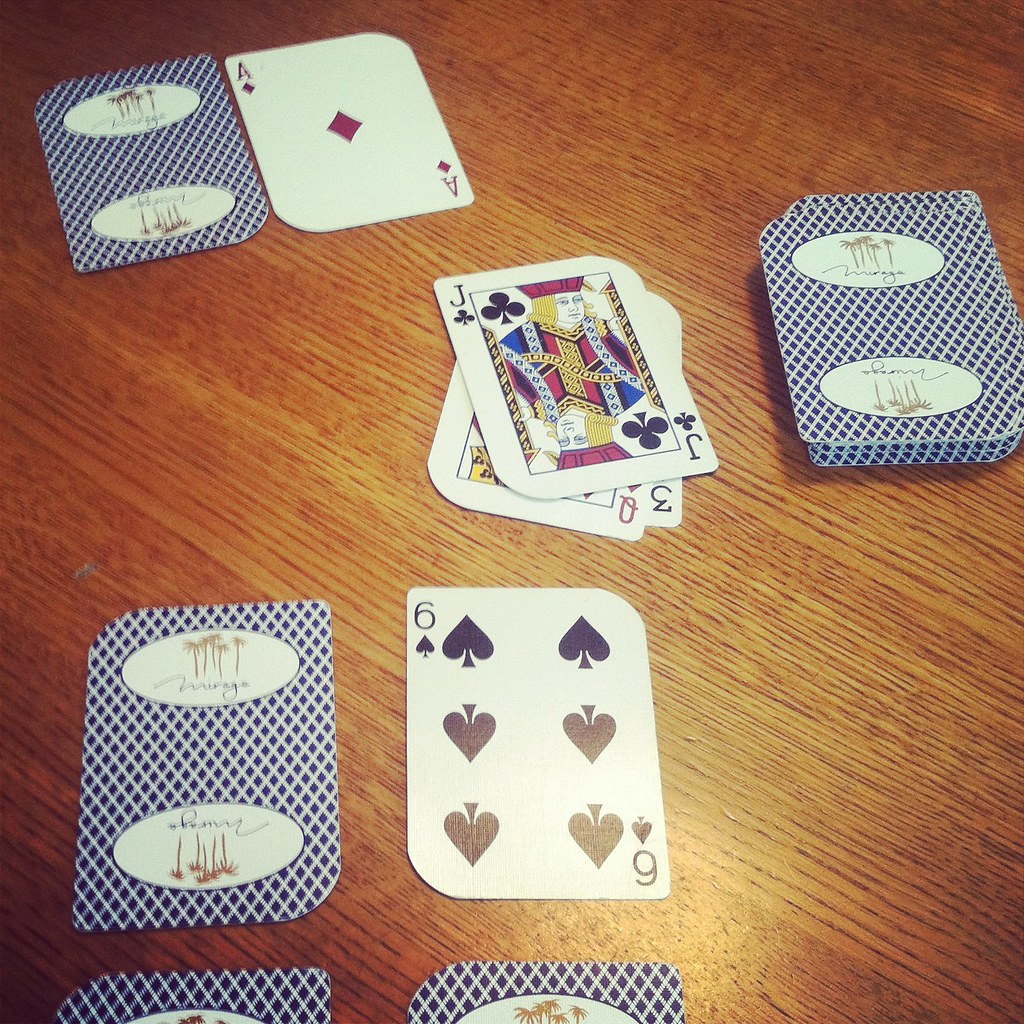On a warm, golden brown wooden table, a collection of playing cards is laid out with a blend of face-up and face-down cards. The cards are notable for their distinctive design: the lower left and upper right corners are significantly more rounded compared to the slight curves on the other two corners. Their large-print symbols make them easily readable, enhancing their visual appeal. The backs of the cards feature a captivating pattern of blue diamonds against a white background, or conversely, white crosshatches on a blue background. A golden silhouette of five palm trees and the scripted name "Mirage" adorn the back of each card, hinting at possible casino origins.

From top to bottom, the image reveals a face-down card followed by an ace of diamonds face-up. Moving down, a jack of spades is seen slightly overlapping a queen of hearts (or diamonds) and a black three. To their right lies a partial deck of undealt cards. As we progress further down, another pair of up and down cards comes into view, with the six of spades positioned on the right. Finally, at the bottom of the image, the card backs of two additional cards are visible. The overall arrangement offers a snapshot of a game in progress or perhaps one that has just concluded.